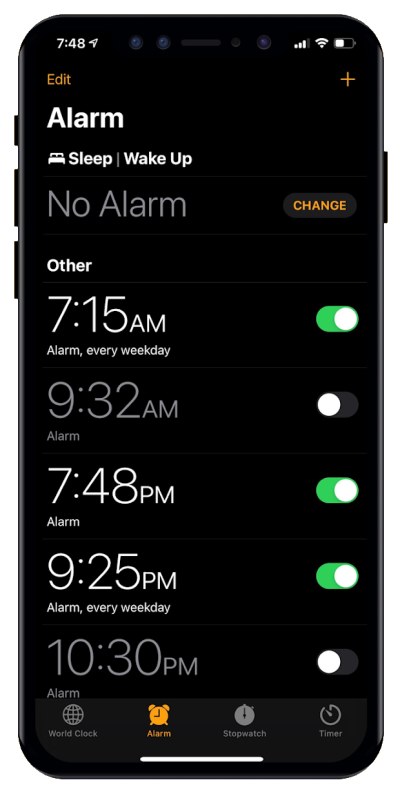The image depicts a smartphone screen displaying the alarm clock interface. At the top, the status bar shows the current time, Wi-Fi signal strength, and battery percentage. Below this are various controls: an orange "Edit" button, an orange "+" sign, and further down, an alarm section labeled "Sleep" featuring a bed icon, with an option marked "Wake Up" indicating no set alarm. An orange "Change" button is also present beneath this.

In the "Other" section, a list of alarms is visible. The first alarm is set for 7:15 a.m. on weekdays, which is active, denoted by a green indicator. A 9:32 a.m. alarm is shown in gray, indicating it is inactive. The third alarm shows a 7:48 p.m. setting, marked as active with a green indicator. Another active alarm is set for 9:25 p.m. on weekdays, signified by a green circle. The final alarm, set for 10:30 p.m., is displayed in gray, indicating it is turned off.

At the bottom, there are navigation tabs: "World Clock" with a globe icon, "Alarm" highlighted in orange, "Stopwatch" symbolized by a clock icon, and "Timer" denoted by a timing device icon.